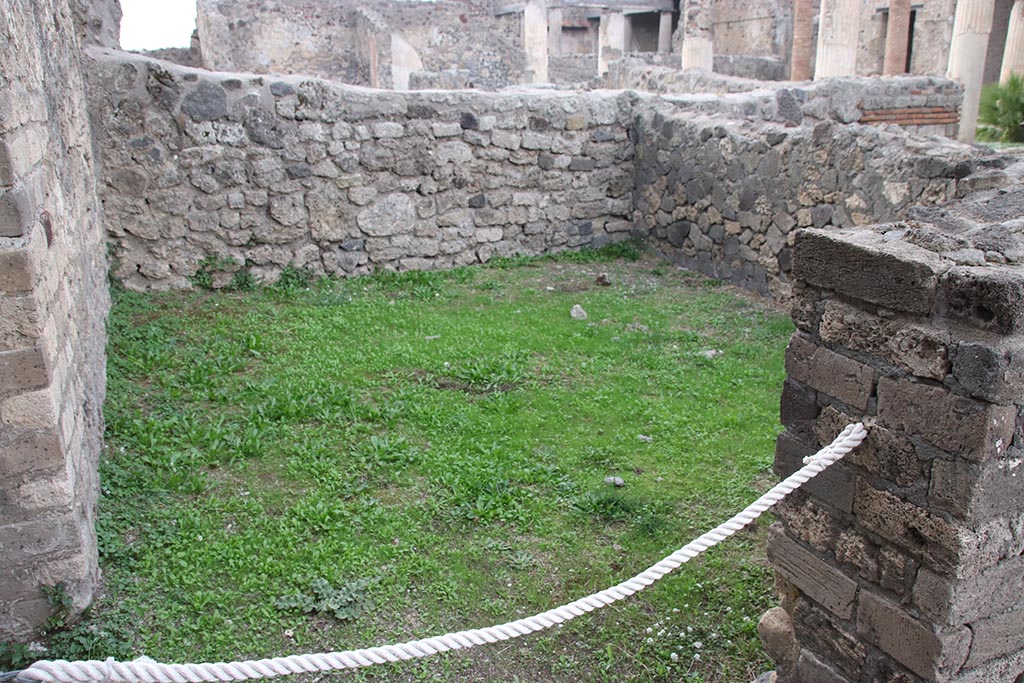This black and white image captures the remnants of a large, ancient building, resembling those found in European cities such as Rome. The structure appears heavily damaged, possibly from war, with a tall wall extending from the bottom right corner towards the middle left side of the image. Lining this wall and prominently featured are numerous broken columns, each reduced to stubs about three feet high. Behind the wall, a labyrinth of rooms is visible, most lacking roofs and consisting of partial walls interspersed with rubble and fallen bricks. The layout suggests foundations of old homes or buildings that have collapsed over time, some still bearing remnants of clay tile roofs. In the foreground, tiny figures can be seen near the wall's base, though their identities and actions are unclear due to the image's scale. The overall scene conveys a sense of historical devastation and the enduring legacy of a once grand architectural site now left in ruins.